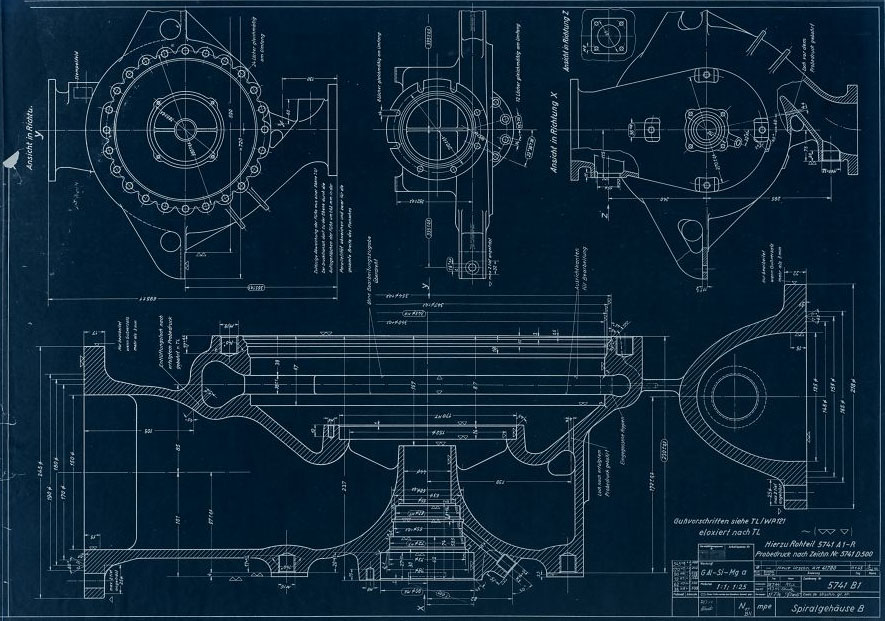This rectangular image, approximately six inches wide and four inches high, showcases a detailed blueprint sketch, predominantly rendered in white on a dark blue background. The blueprint appears to be an engineer or architect's illustration of an intricate device, comprising multiple gears and components. The border of the image features a thin light blue line, tracing from the upper left corner to the right, then down to the lower right, moving left to the lower left, and finally, back up towards the starting point, stopping about 3 1/4 inches from the upper left corner.

The top section of the blueprint is divided into three distinct diagrams: 
1. On the left, a triple-layered circle resembling a chain encompassing a smaller circle, with metal parts extending outwards.
2. In the center, a smaller, plain circle.
3. On the right, a semi-circle with a vertical piece attached, reminiscent of a cannon shape. Adjacent to this is another diagram on the upper right with a cannon-like shape pointing leftwards.

The lower half of the blueprint features a prominent sketch extending horizontally across the top, showcasing long horizontal lines and a slender base that widens as it descends. 

The entire layout is meticulously annotated with specifications and dimensions, though the text is too small to discern exact details. Both the upper left and lower right corners contain foreign language text, with the bottom right bearing the words "Spiral Gay House" (S-P-I-R-A-L-G-E-H-A-U-S-E), providing an additional hint towards the design’s potential origin.

The overall impression is that of a highly detailed and technical digital print, explaining various parts of an unknown device.